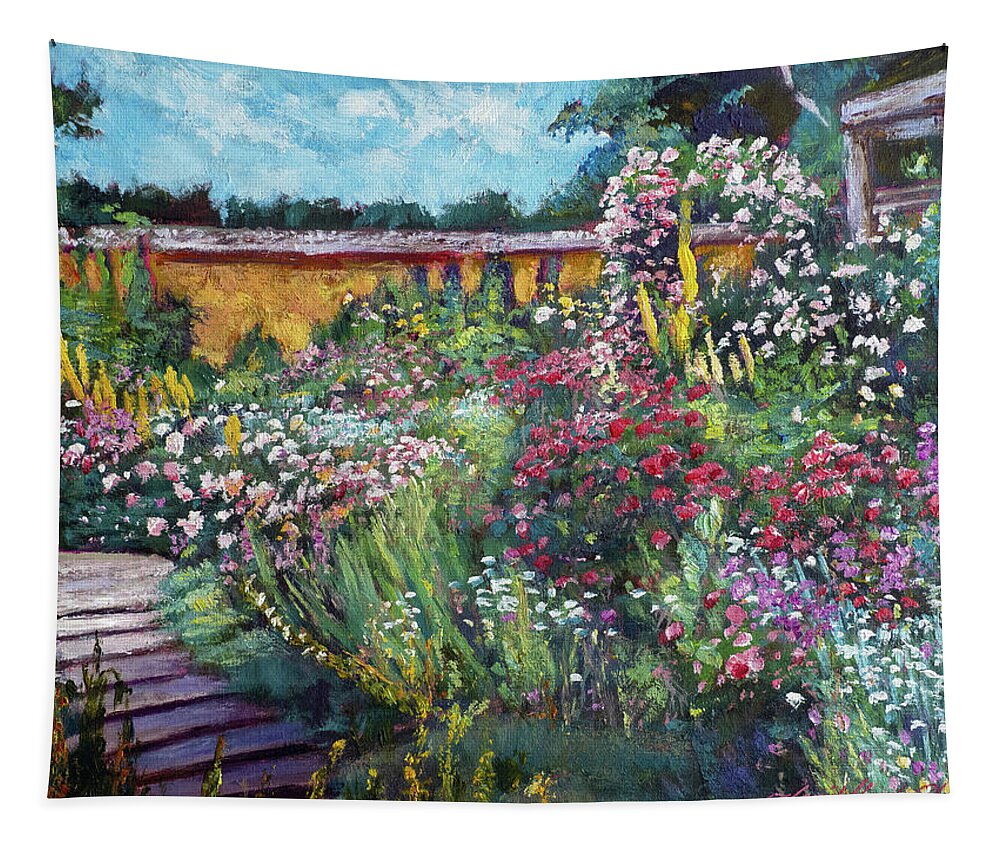The image depicts a lush and vibrant garden captured in a painting, likely printed on a cloth banner as indicated by the uneven sides. The scene is an explosion of colors, with red, pink, white, purple, and yellow flowers dominating the landscape. The garden appears very dense with greenery and blossoms, creating a rich and full visual experience. In the lower left-hand corner, stone steps emerge, partially overgrown with grass. In the middle ground, there is a yellow border-like structure that separates the garden from a stretch of trees in the background. Above, the blue sky is dotted with white clouds, providing a serene backdrop to the vivid floral display. The combination of various flowers, detailed stonework, and a picturesque sky makes this painting a captivating and well-executed depiction of a beautiful outdoor garden scene.